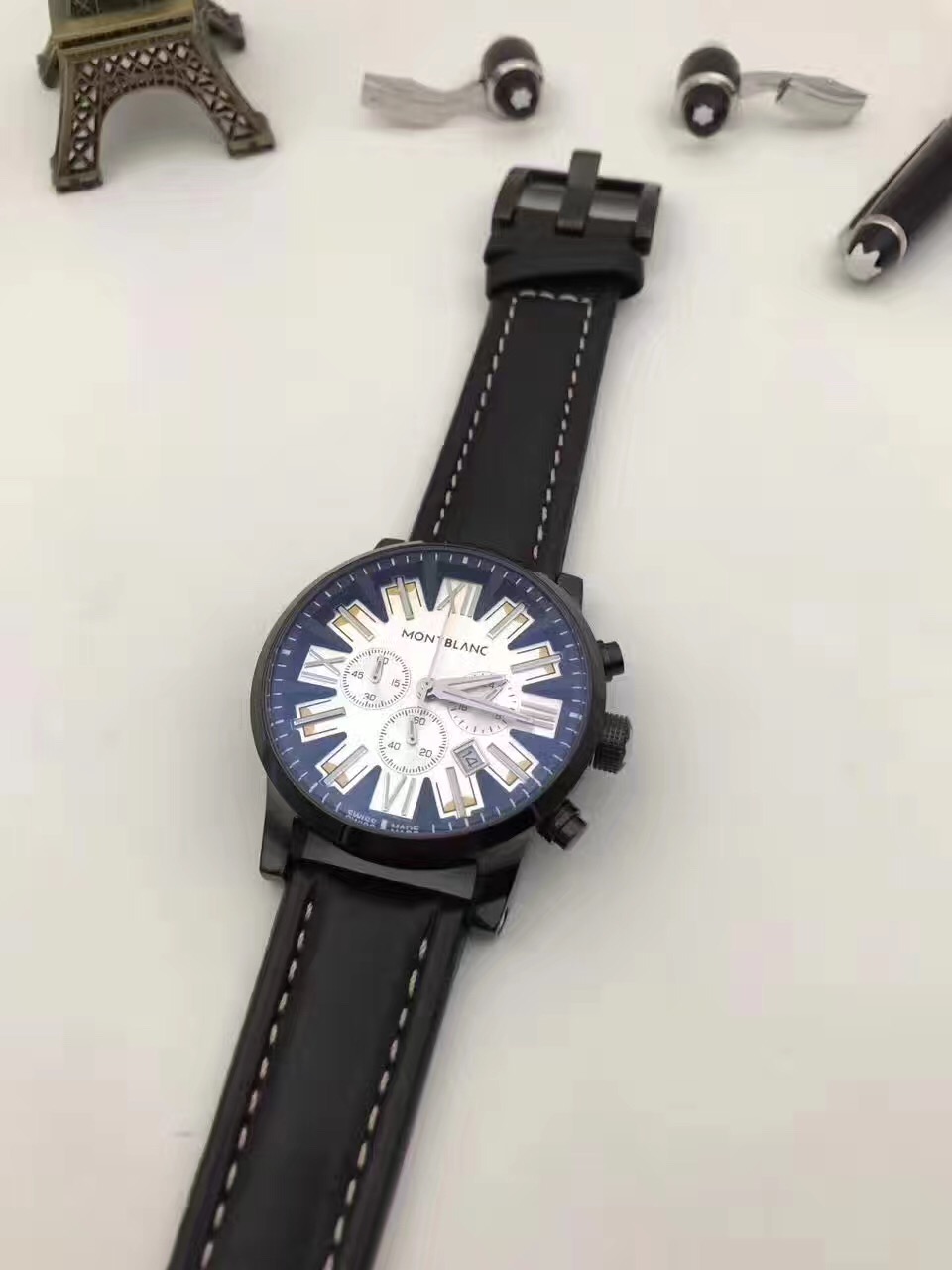A meticulously styled Montblanc wristwatch is showcased against a white background, subtly adorned with objects at the top portion. The watch features a black leather strap that exudes sophistication. The face of the watch is a striking combination of blue and white, with the iconic Montblanc name elegantly printed in black letters at the top. Complementing the face are sleek silver hands indicating a time of approximately 2:16, accompanied by additional second hands for precise timekeeping. In the upper section of the image, the bottom part of a miniature Eiffel Tower can be seen, with two metal clips positioned slightly above it. Just above these, to the right, lies a pen cap, adding an intriguing layer of context to the composition.